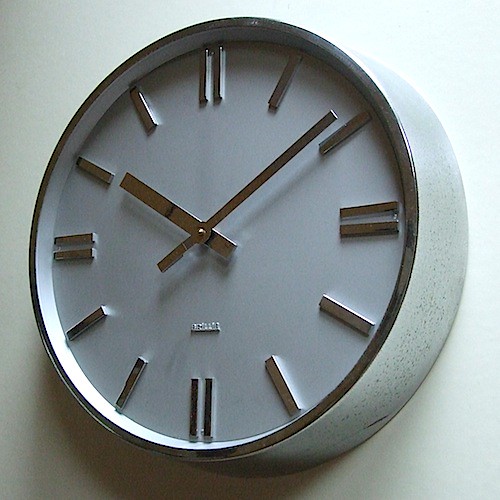A sleek, modern wall clock design is showcased in this image. The clock is predominantly gray with a striking black edge that adds a touch of elegance. Instead of traditional Roman numerals, the clock features minimalistic black slats, with two slats marking the 12, 3, 6, and 9 positions, and single slats indicating the other hours. The clock's hands follow the same modern, geometric slat design, creating a cohesive aesthetic. Additionally, the manufacturer's name is embossed in gray between the center and the 6 o'clock position, though it is not legible in the image.